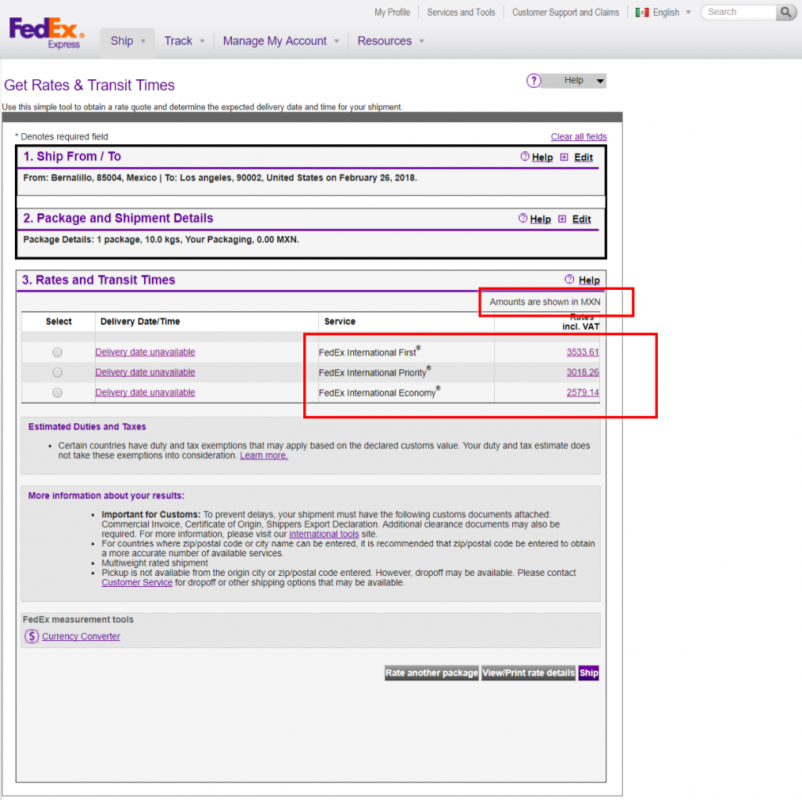A screenshot of a FedEx Express webpage. The top section has a prominent navigation bar featuring the FedEx logo on the far left, followed by tabs for "Ship," "Track," "Manage Account," and "Resources." Under these tabs, additional options are accessible, such as "My Profile," "Services and Tools," and "Customer Support," along with a search bar. Below the navigation bar, the page is focused on shipping features. It displays a menu to "Get Rates and Transit Time," followed by a blank shipment information form labeled "Ship From" and "Ship To." This form is centrally located and bordered in red. The right side of the form seems to have fields for "Delivery Time" and accompanying details. Further down, there are sections presumably for inputting amounts (shown in a currency, possibly MXN). Additional features like a currency converter and other shipping-related tools are available towards the bottom of the screen.